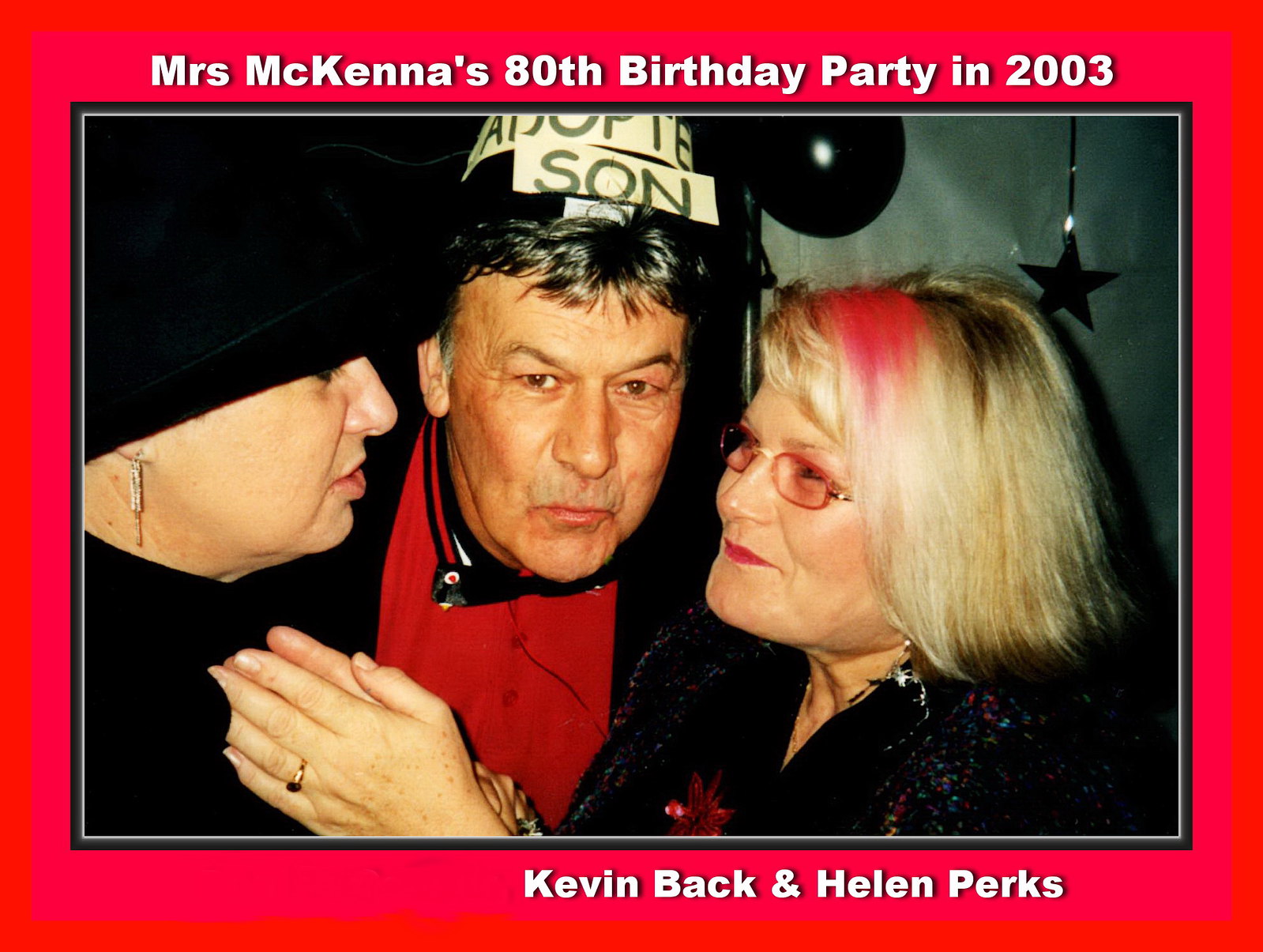The close-up image captures three individuals, with an older man positioned centrally, likely in his 50s or 60s. He's adorned with a hat that has the words "Adopted Son" on it and appears to be puckering his lips. Flanking him are two women, both seemingly older as well. The woman on his right is dressed entirely in black, including a black hat and earrings, and she is staring directly at the other woman. The woman to his left has blonde hair with a pink stripe, red glasses, red lipstick, and wears a sparkly black shirt. She is gesturing towards the woman on the right. A star decoration hangs from the ceiling amid a dark background, suggesting a festive occasion. The image features a flat red border with white text that reads: “Mrs. McKenna's 80th birthday party in 2003 - Kevin Beck and Helen Perks.” Bright red and predominantly party-themed, the photograph conveys a celebratory atmosphere.